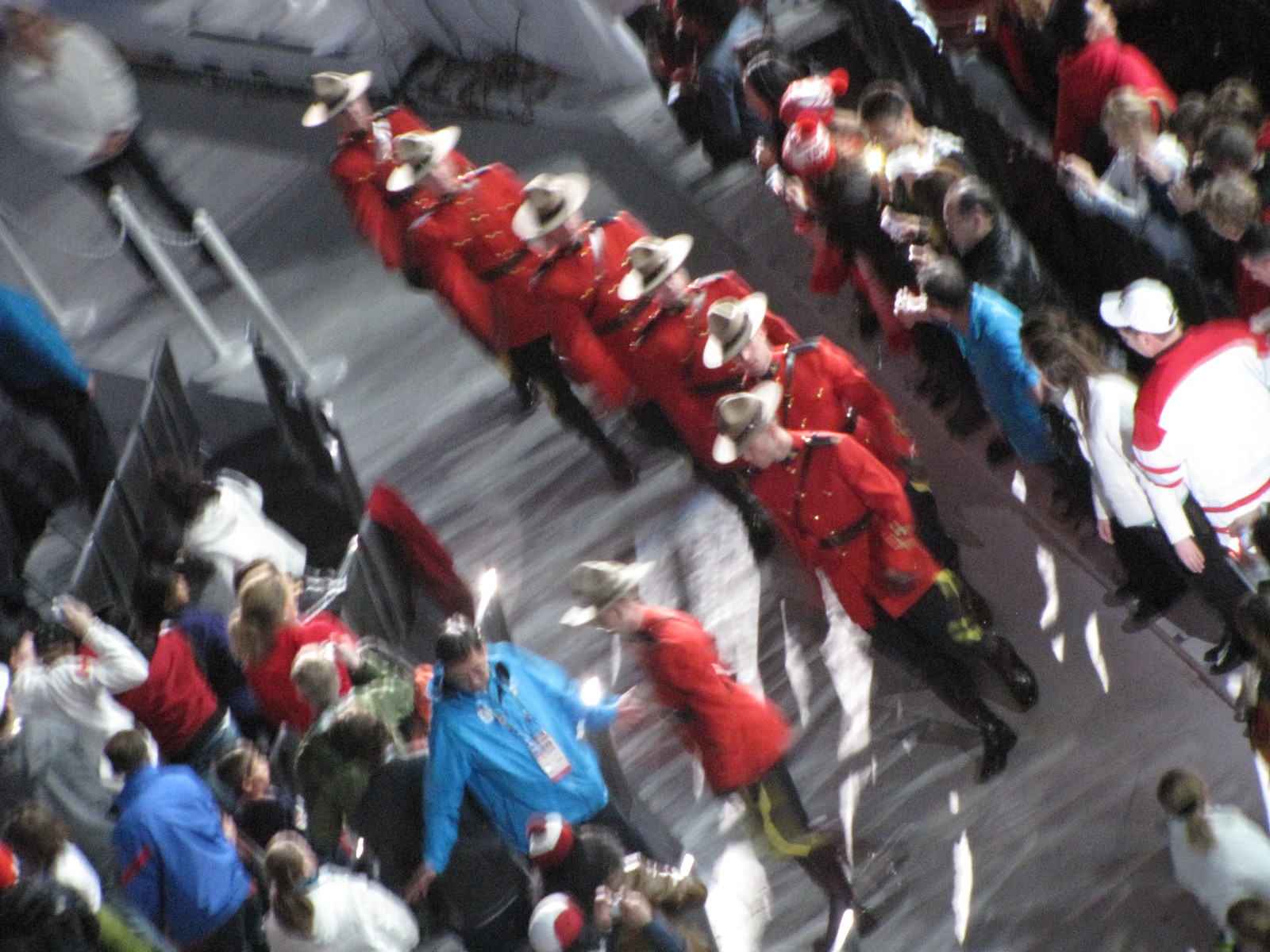This blurred, top-down photograph captures a procession of nine or ten Canadian Mounties in uniform, taken at an indoor event. The Mounties, easily recognizable by their wide-brimmed tan hats with brown leather straps, are marching in a line from the top left towards the center of the image. They're dressed in traditional red jackets adorned with brass buttons, black pants featuring two yellow stripes down the sides, black gloves, and black boots. Their distinctive uniform also includes a strap running diagonally across their chest. The event appears to be a hockey game, evidenced by spectators wearing hockey jerseys, including a man in a white and red jersey with a white baseball cap. In the bottom left, a Mountie is seen slightly out of formation, moving towards the crowd, seemingly directed by a person in a blue jacket, possibly a stadium staff member. Surrounding the Mounties, people are lined up along the aisles on a gray cement floor. Despite the image's poor quality and noticeable motion blur, the scene vividly depicts the orderly procession of the Mounties in this bustling indoor setting.